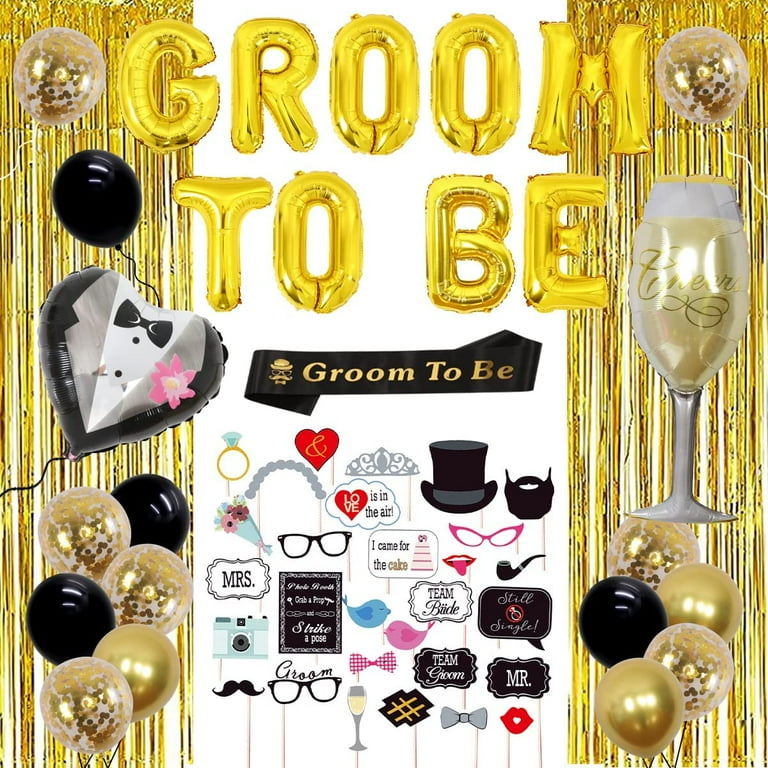The promotional advertisement showcases an array of novelty items for a groom-to-be, ideal for a bachelor or pre-wedding party. Dominating the top of the ad are large golden letter-shaped helium balloons spelling out "GROOM TO BE," complemented by black, white, gold, and silver party balloons and streamers. A distinctive black ribbon banner, also inscribed with "GROOM TO BE" in gold lettering, hangs beneath. The scene is festively adorned with gold tinsel and other decorative elements. Among the items displayed are a wine glass labeled "GROOM," numerous clip-art-style party props such as top hats, moustaches, glasses, and lips on sticks. Various signage offers playful messages like "Mr.," "Mrs.," "Team Groom," "Team Bride," and "Love is in the Air," along with humorous notes like "I came for the cake." Additional thematic elements include a tuxedo balloon and a wine glass balloon inscribed with "Cheers." The image’s cohesive use of gold with accenting black and white underscores an elegant yet whimsical celebration atmosphere.